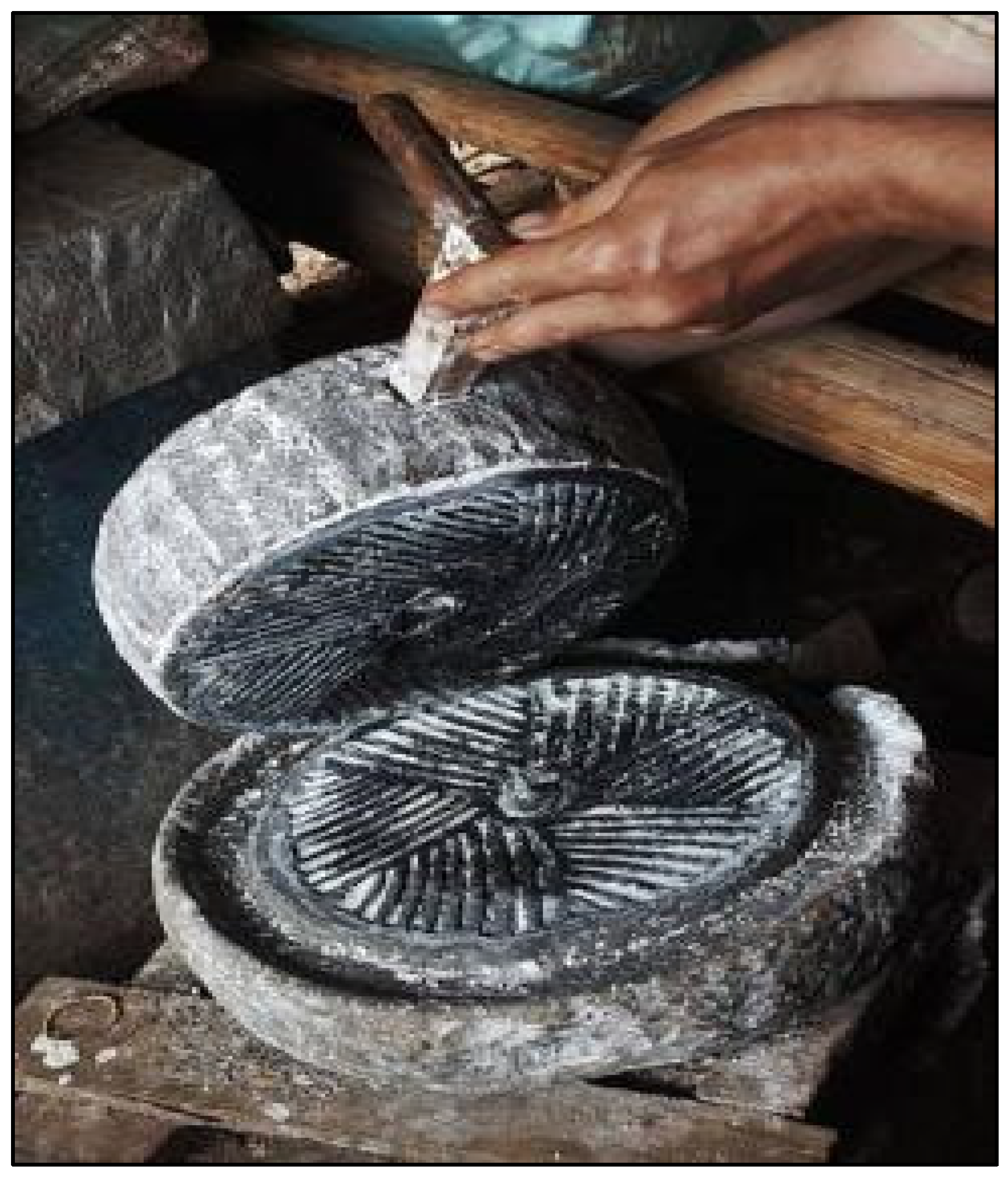The color photograph features a close-up of an ancient stone grinding mill. The mill comprises two circular granite stones, a base stone and a top stone, both with interlocking grooves for effective grinding. The top stone, fashioned with a handle, is being lifted by a person with dark brown skin whose hands are the only visible part in the image. The grinder rests on a simple wooden frame against a background that includes dried-out bamboo or wooden beams, as well as small stone slabs in the top left corner. The mill's granite stones are a deep gray color, and there is a rimmed edge around the bottom stone to catch the ground material, with a mechanism at the back to pour it off.